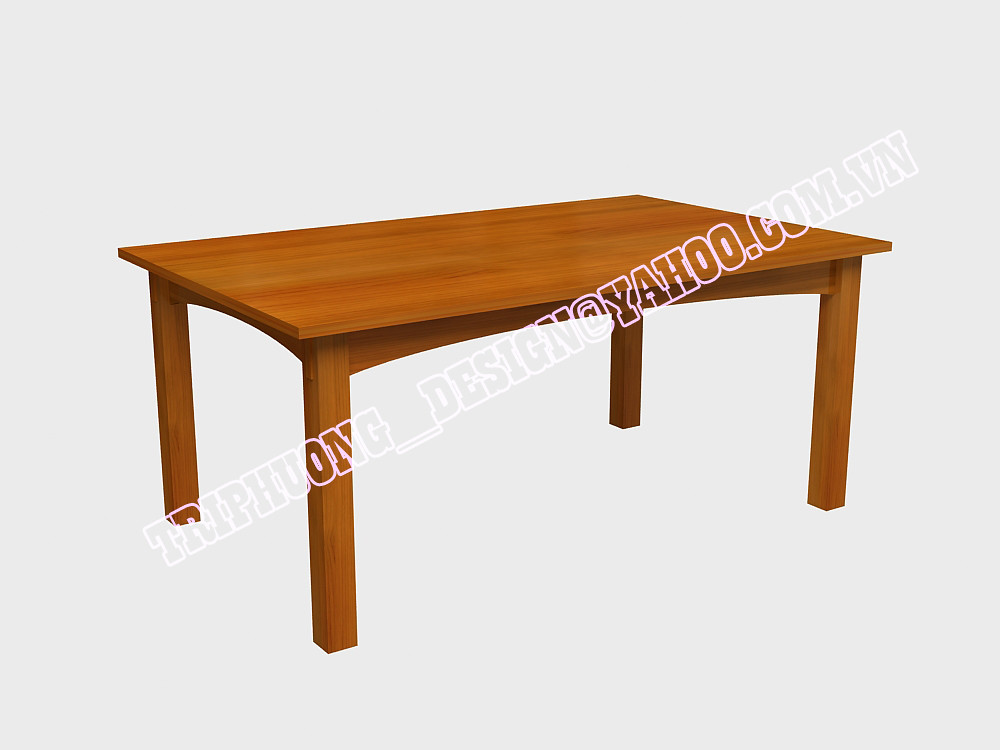This is a computer-generated stock image of a medium-brown wooden table set against a white background. The table, featuring a rectangular shape, is angled with the right side pointing slightly upwards towards the top right corner of the image. It has four legs, supported by a slightly arch-shaped beam that connects the top parts of the legs beneath the tabletop. Overlaid diagonally across the center of the image is the text "triphuong_design@yahoo.com.vn" in purple lettering, with a pink border around the transparent text.